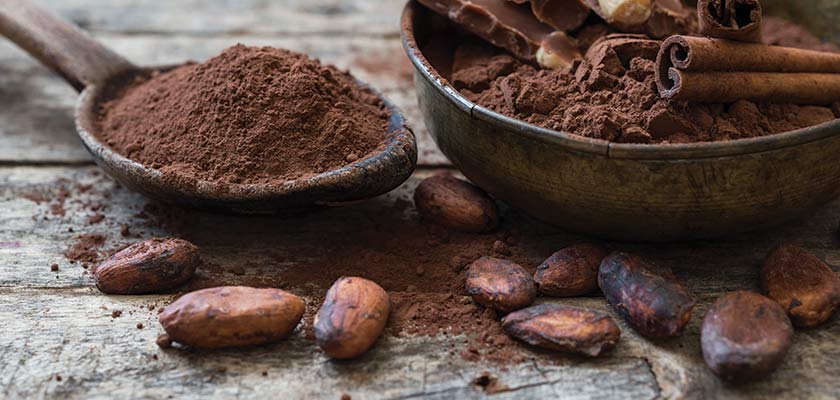This high-definition image, likely taken by a food blogger, showcases a rustic, weathered gray wooden table. On it rests a worn and broken metal bowl, possibly made of copper with a dark gray hue and visible damage. The bowl is filled with rich, finely ground cocoa powder, and interspersed with whole cocoa beans, ranging in color from light brown to dark brown, and resembling the shape of almonds.

A wooden spoon with a dark-grained wooden handle lies to the upper left side of the photo, also containing cocoa powder. Scattered around the bowl and spoon are more cocoa beans and sprinkles of cocoa powder, adding to the composition’s raw and earthy aesthetic.

The light source is natural, illuminating the table and its contents, highlighting details such as the table's scratches and wear. Additional elements include a dark chocolate bar with white nuts, a cinnamon stick, and potentially a chocolate wafer, enhancing the image’s rich and inviting presentation of cocoa in its various forms.